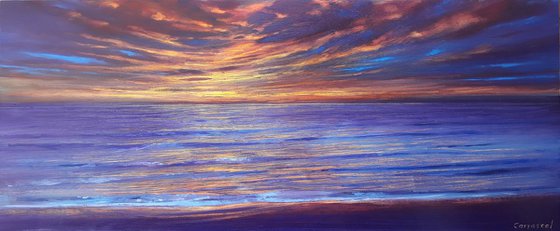The image depicts an artistic rendition of a sunset over the ocean, set against a white background. The top portion of the rectangular scene features a bright blue sky, transitioning into hues of yellow and gold to illustrate the setting sun. The sky, rippled with orange clouds and backlit by the sun, gradually merges with the blue sea below.

The ocean, filled with varying shades of blue, displays a glistening reflection of the sunset, with areas in the middle painted with yellows and oranges. These reflections add a warm glow, creating a serene and calm atmosphere. At the bottom of the picture, the beach is depicted with purplish dark colors, contrasting with the brighter hues of the water and sky.

An orange horizon seamlessly connects the sky and sea, while the waves near the shore are tinged with gold. The beach's sand appears dark, almost black at the bottom, shading into gold as it approaches the water.

The overall composition beautifully captures the transition of colors from a golden sunset to the calming blues of the ocean, with a signed signature in a translucent white font at the bottom right, partially faded and starting with the letter 'C.'